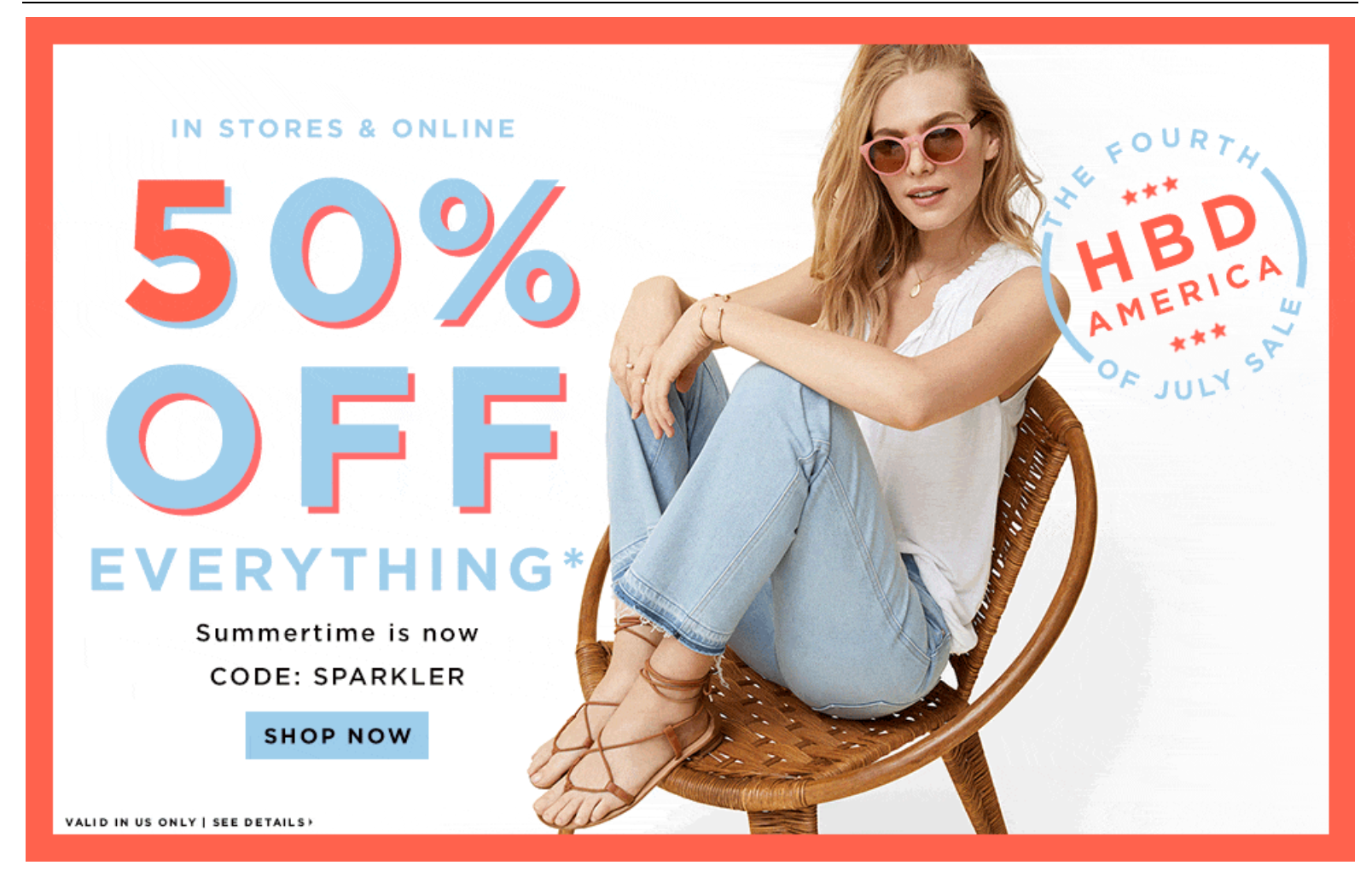This is a detailed caption for the described image:

The advertisement screenshot features a strikingly detailed layout. At the top of the image, there's a black vertical bar intersected by a black horizontal bar. The entire advertisement is bordered in red, while the center remains a pristine white. Centrally placed within this white background is a photograph of a woman exuding casual elegance. She is a white woman with blonde hair, styled in a relaxed manner. She dons round sunglasses and has her mouth slightly parted, revealing her white front teeth. Her accessories include a golden necklace with a locket, multiple bracelets adorning her wrists, and several rings on her fingers.

The woman is comfortably seated in an egg-shaped wicker chair, with her feet propped up, causing her arms to rest on her knees. Her attire includes a white tank top paired with light blue jeans and brown sandals. Notably, her sandals hint at a festive touch with small bells attached to them. 

To the right of the woman, there is a prominent insignia proclaiming, "4th of July Sale - HBD America". On the opposite side, to her left, bold text announces, "In stores and online - 50% off everything", followed by an asterisk indicating that certain exclusions apply. Below this is a cheerful summer slogan, "Summertime is now! Code: Cohen Sparkler. Shop Now". The composition of the advertisement is visually appealing and effectively conveys a festive, celebratory atmosphere.